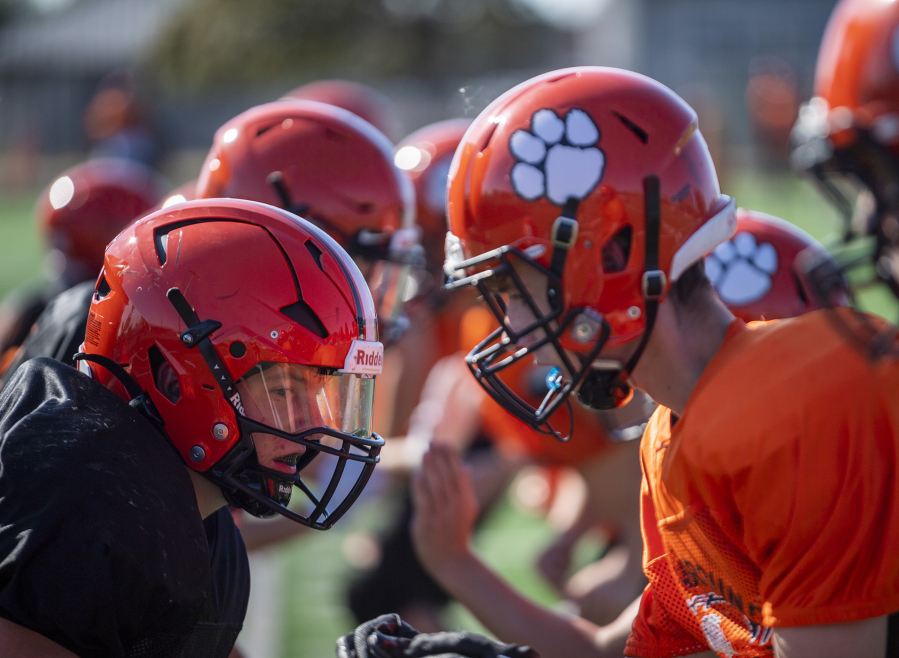In this detailed photograph, two young teenage football players are seen facing off on a field, likely in a high school or middle school game. The Clemson player on the right, slightly taller, is donning an orange jersey with a red helmet emblazoned with a distinctive white paw print. Directly opposite him, a player from the opposing team wears a black jersey with a red helmet that has a black design. The intensity of the moment is captured as these two focused players, both clearly in the foreground, prepare for a play. A blurred background shows more players lined up, adding depth to the scene. The arm of another player is seen reaching up between the two central figures, hinting at the anticipation of the game's kickoff or a play's initiation. The background hints at the surroundings of a typical football field, although details remain indistinct due to the blur.